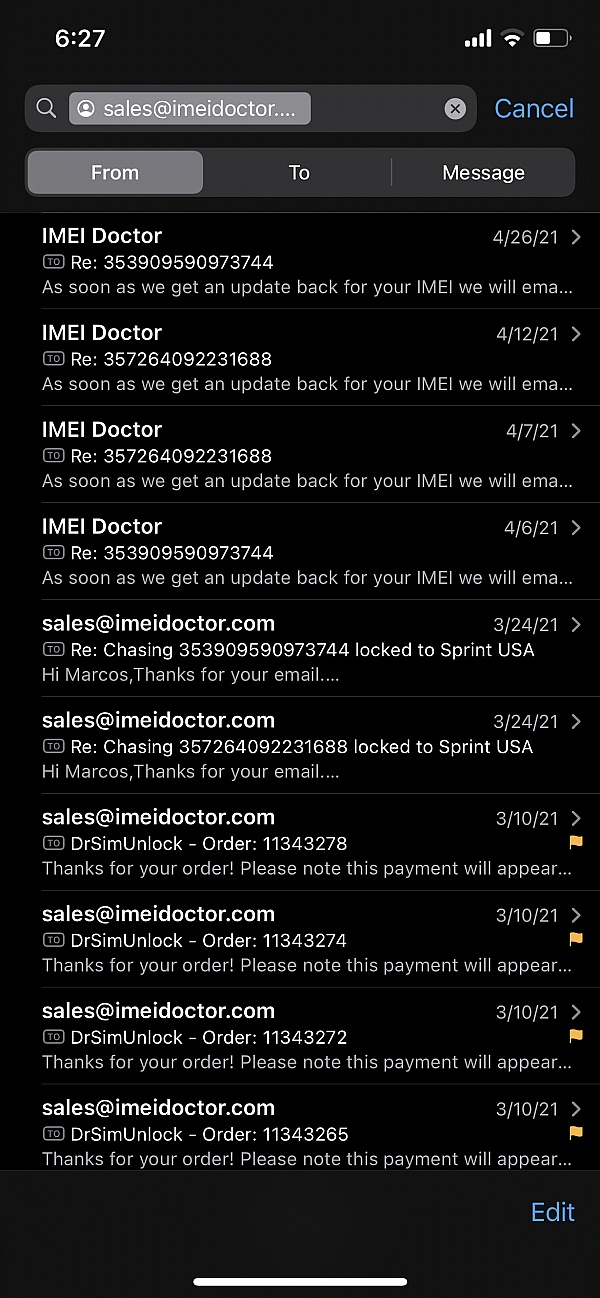This image captures a screenshot of an email inbox on an iPhone. The phone is displaying dark mode, rendering the screen predominantly black with white text. The status bar at the top indicates it is 6:27 PM, the device is connected to Wi-Fi with full cellular signal strength, and the battery is approximately 50% charged. The user is actively searching their email for correspondences from "sales@IMEIdoctor." The inbox reveals numerous email threads, each with subject lines containing miscellaneous numbers, suggesting follow-up communications. The emails originate from "IMEI Doctor" and "sales@IMEIdoctor," with some also referencing "Doctor SIM Unlock." These messages date back to March and April 2021 and seem to be related to orders for SIM cards or mobile services, possibly linked to a Sprint USA cell phone plan. The majority of the screen is filled with these email interactions, painted in stark black and white hues.